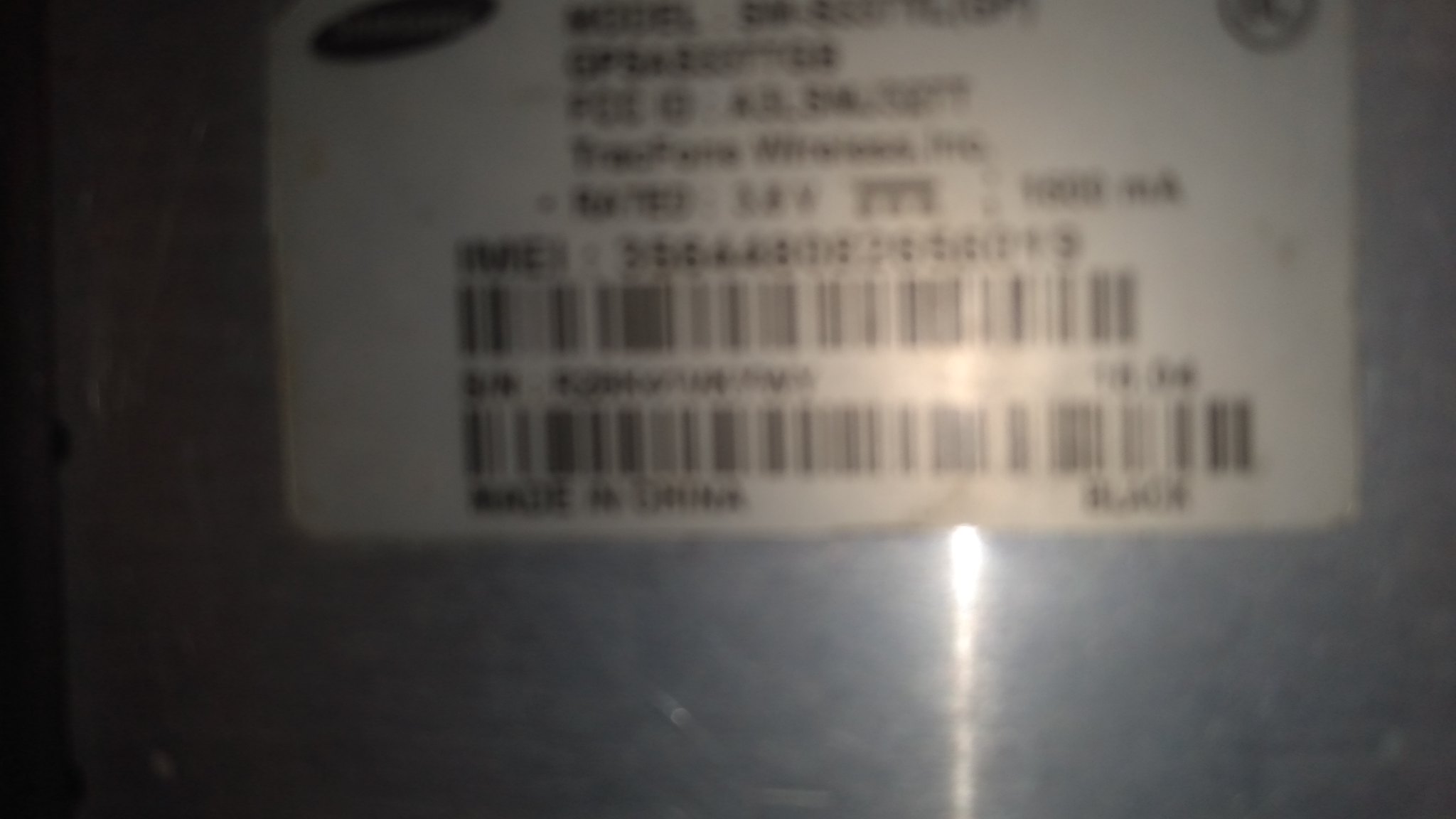The photograph showcases a white label, resembling a sticker, affixed to a silver metal surface, possibly the back or bottom of an electronic device like a computer tower. The image is taken in a dark room with the label illuminated by a light source, causing a bit of light reflection. Despite the scene being well-lit, the photograph suffers from significant motion blur, rendering the text and barcodes on the label unreadable. The label displays an IMEI number, various serial numbers, and two distinct barcodes, positioned with one at the bottom of the label. The text and all symbols on the sticker are in black, but they remain obscured due to the blurry effect, similar to viewing without glasses. Additionally, "Made in China" appears to be printed at the bottom.